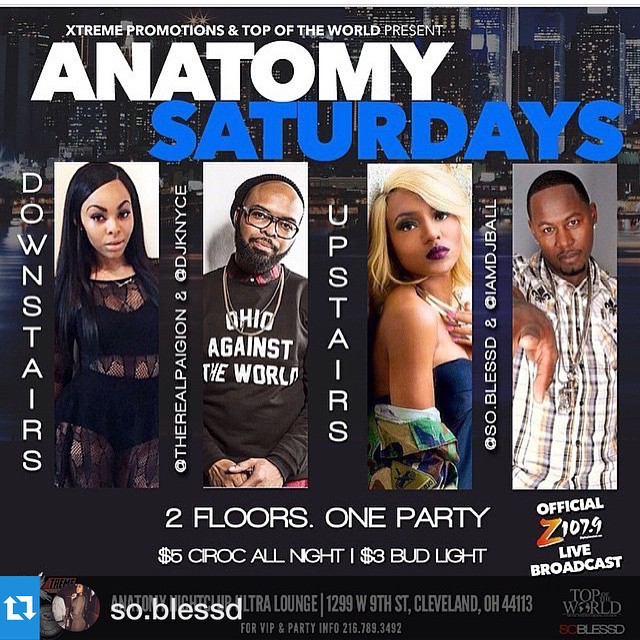This detailed advertisement poster for an event hosted by Extreme Promotions and Top of the World presents a vivid and dynamic nightlife experience at Anatomy Nightclub Ultra Lounge. The nighttime city skyline forms a sleek black background, accentuating the white, bold all-caps text at the top. In substantial white letters, the event is titled "ANATOMY" with "Saturdays" prominently highlighted in bold blue beneath it. 

The layout features images of four individuals, each accompanied by their stage names and roles. On the left, under the title "Downstairs," is a woman with dark hair and the names "The Real Payon" and "DJ Cave." Next to her, under the title "Upstairs," is a blonde woman labeled "Upstairs" with "So Blessed" and "I Am DJ Ball." A male figure with glasses also appears with the title "DJ Nice". 

Below the images and setting details are promotional highlights: "Two Floors, One Party," and pricing information including "Five Dollar Crock All Night" and "Three Dollar Bud Light." The bottom of the poster prominently includes "Official Z 107.9 Live Broadcast."

For those interested in more details or VIP access, the address "1299 West 9th Street, Cleveland, Ohio 44113" and contact number "216-789-3492" are provided, ensuring that all potential attendees have the necessary information to join the event.